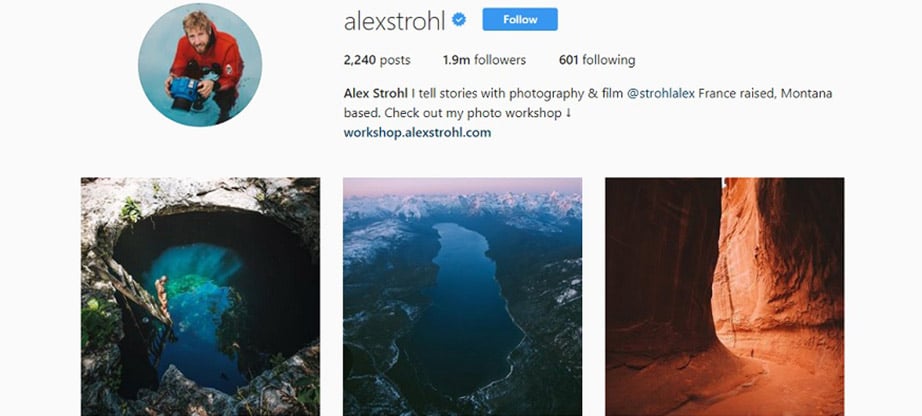This image is a detailed screenshot from the Instagram account of Alex Strohl, identifiable as @alexstrohl, who has a verified blue checkmark next to his name. The profile features a circular thumbnail on the left, showing Alex dressed in a red jacket, holding an underwater camera, with dirty blonde hair and a matching beard. His account details indicate he has posted 2,240 times, amassed 1.9 million followers, and follows 601 accounts.

Beneath his name, his bio reads: "Alex Strohl. I tell stories with photography and film at Strohl Alex. France-raised, Montana-based. Check out my photo workshop: workshop.alexstrohl.com."

Directly below the bio, three aesthetically striking landscape photographs are displayed side by side. The first image on the left captures a person diving into a brilliantly blue and green swimming hole, which is carved out of rock, reminiscent of a cave. The center photograph showcases a serene river, flanked by majestic mountains capped with pristine white snow. The final image on the right depicts towering red rock formations in a desert, with a pathway winding between them. Each photograph highlights Alex's keen eye for natural beauty and adventure photography.